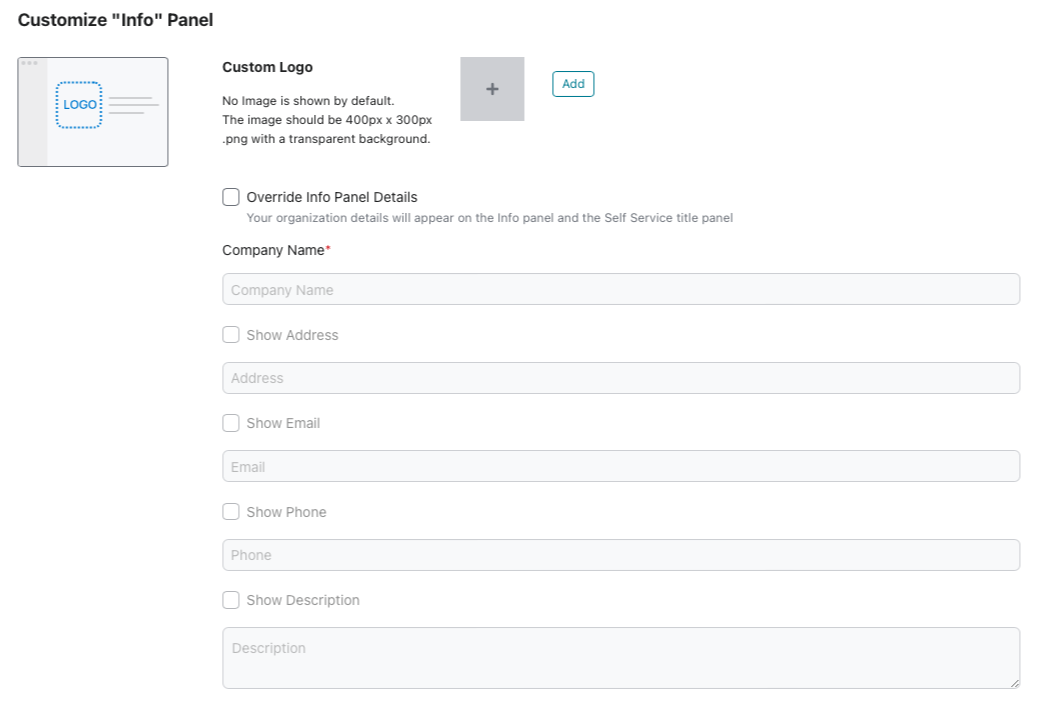In the image, there is a webpage interface specifically for customizing various elements of an info panel. The main section on the left prominently features a text header that reads "Customize Info Panel," alongside options for incorporating a custom logo. This section does not display any images by default, but it specifies that the image to be added should be 400 pixels by 400 pixels in dimension and preferably in PNG format with a transparent background for optimal integration.

Adjacent to this main section, on the right, is a designated field where users can upload their PNG images. The interface encourages users to click this field to add images, making the customization process straightforward.

Below these primary sections, there are additional configuration options. One such option labeled "Override Info Panel Details" is currently unchecked, which implies that the default organization details will be displayed on both the info panel and the self-service title panel. Several fields beneath this include placeholders for "Organization Details," "Show Address," "Show Email," "Email," "Phone," and "Description." All of these fields are presently empty, awaiting input from the user to provide comprehensive organization details where applicable.

Overall, the layout is clean and user-friendly, guiding users through the process of personalizing their info panel with minimal effort.